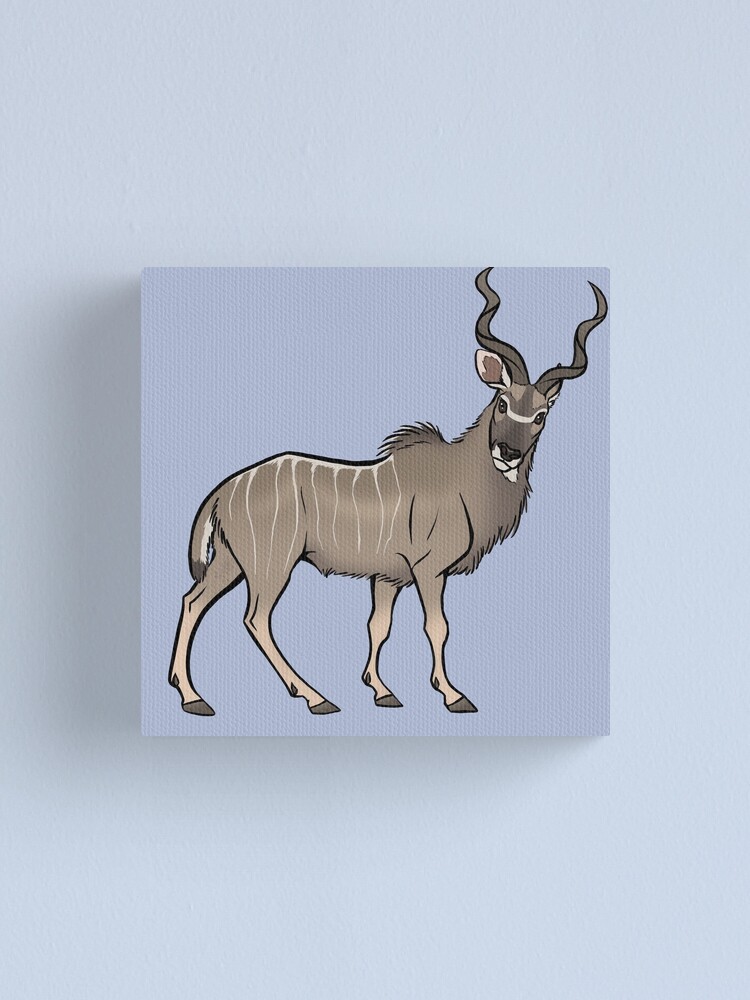The image depicts an art piece painted on a light blue canvas, which is centered against a dull white wall. The painting showcases a majestic antelope-like creature with distinct yet deer-reminiscent features. It is rendered with a rich brown fur, accentuated by white striping along its spine. The creature’s large horns curve gracefully backward rather than branching out like typical antlers. This elegant animal is portrayed in a side view with its head turned, fixing its gaze directly at the viewer. The legs are lighter in color compared to the body, featuring a light brown hue, and the face has touches of white around the tips of the ears and chin. The background within the painting is a solid light blue, which adds a serene contrast to the earthy tones of the antelope.